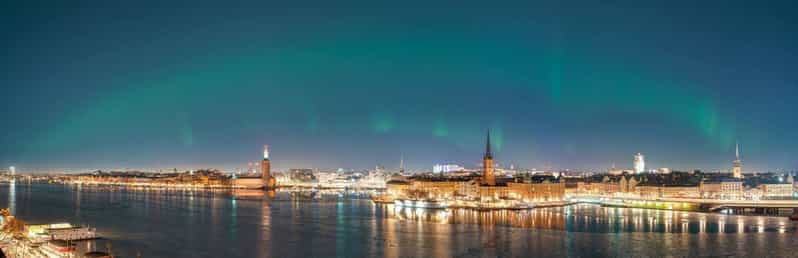The image captures a stunning city skyline under the ethereal glow of the Aurora Borealis. The upper corners of the night sky are a deep blue, transitioning into arches of light teal and bright teal hues, resembling a celestial dance with green, rainbow-like streaks and blotches akin to smoke throughout the sky. Dominating the skyline are several tall buildings, punctuated by sharp, pointed tops. Central among them is a structure with a black spire atop a brown facade. To its left stands another building with a brown base and a white light at its peak, reflected in the waterway that stretches before the city. This water is aglow with the reflections of orange, blue, and white city lights, adding a vibrant shimmer to the scene. The left side of the image features a darker, shadowy bank with a boat dock, while the panoramic view suggests a wide and narrow frame, enhancing the immersive, atmospheric feel of a northern metropolis basking in the aurora's radiant light.